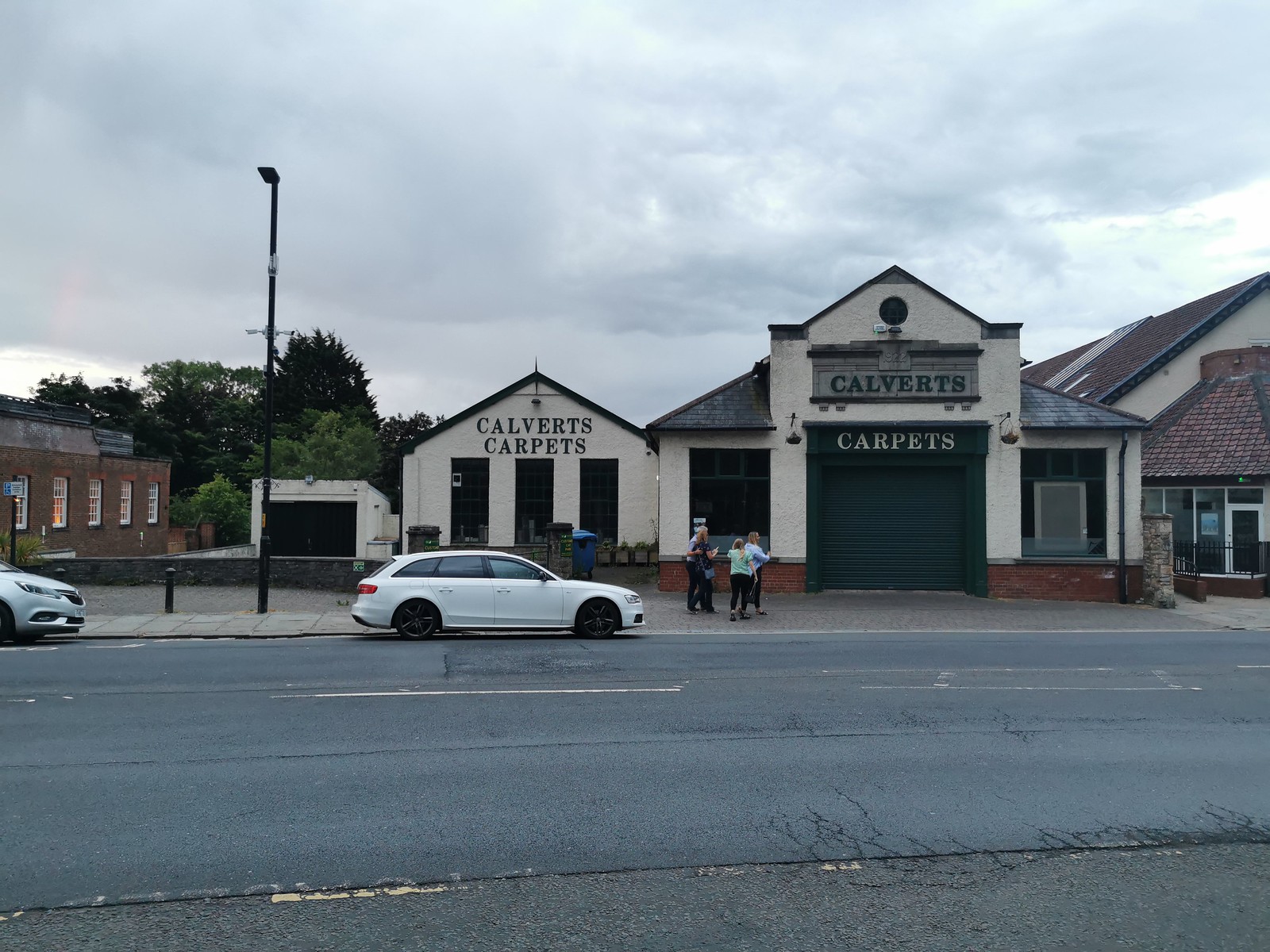This photograph captures an overcast scene with dark, cloudy skies above a street lined with buildings and parked cars. Central to the image is a business named "Calvert's Carpets," which is prominently displayed twice. The business consists of two adjoining one-story buildings, both with peaked roofs. The larger main building features a triangular roof with pillars at the entrance, resembling a residential house or garage. Next to it is a smaller building with either three windows or a combination of windows and doors.

Around the buildings are some light posts and trees. Parked along the street are two cars, one gray and one white. On the sidewalk in front of the business, three people can be seen—two women and one man. All three are wearing black pants; one woman is in a green t-shirt, the other in a long-sleeve blue shirt, and the man in a dark shirt. The whole scene gives off a somewhat dreary atmosphere due to the overcast sky, emphasizing the simplicity and everyday nature of the neighborhood.